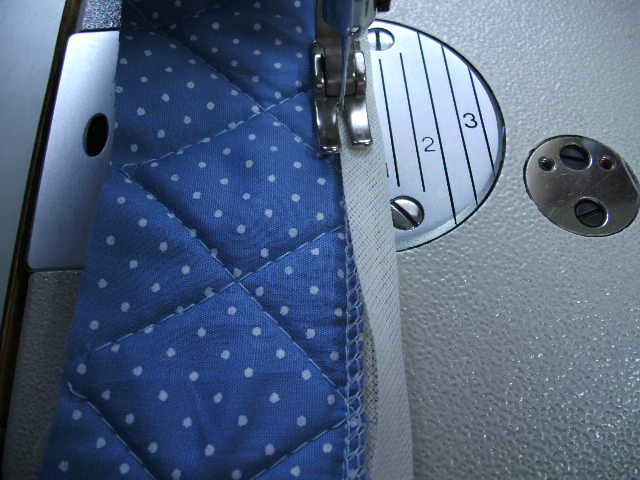The image depicts a sturdy, gray sewing machine in the process of sewing a piece of blue fabric adorned with white polka dots. The fabric, resembling a quilt or perhaps a pot holder, is being stitched along its white edge. Visible beneath the presser foot of the sewing machine are the numbers "2" and "3", along with some metallic circular components and screws. The sewing machine, featuring a bumpy texture, is clearly depicted as a robust and reliable tool for sewing tasks.